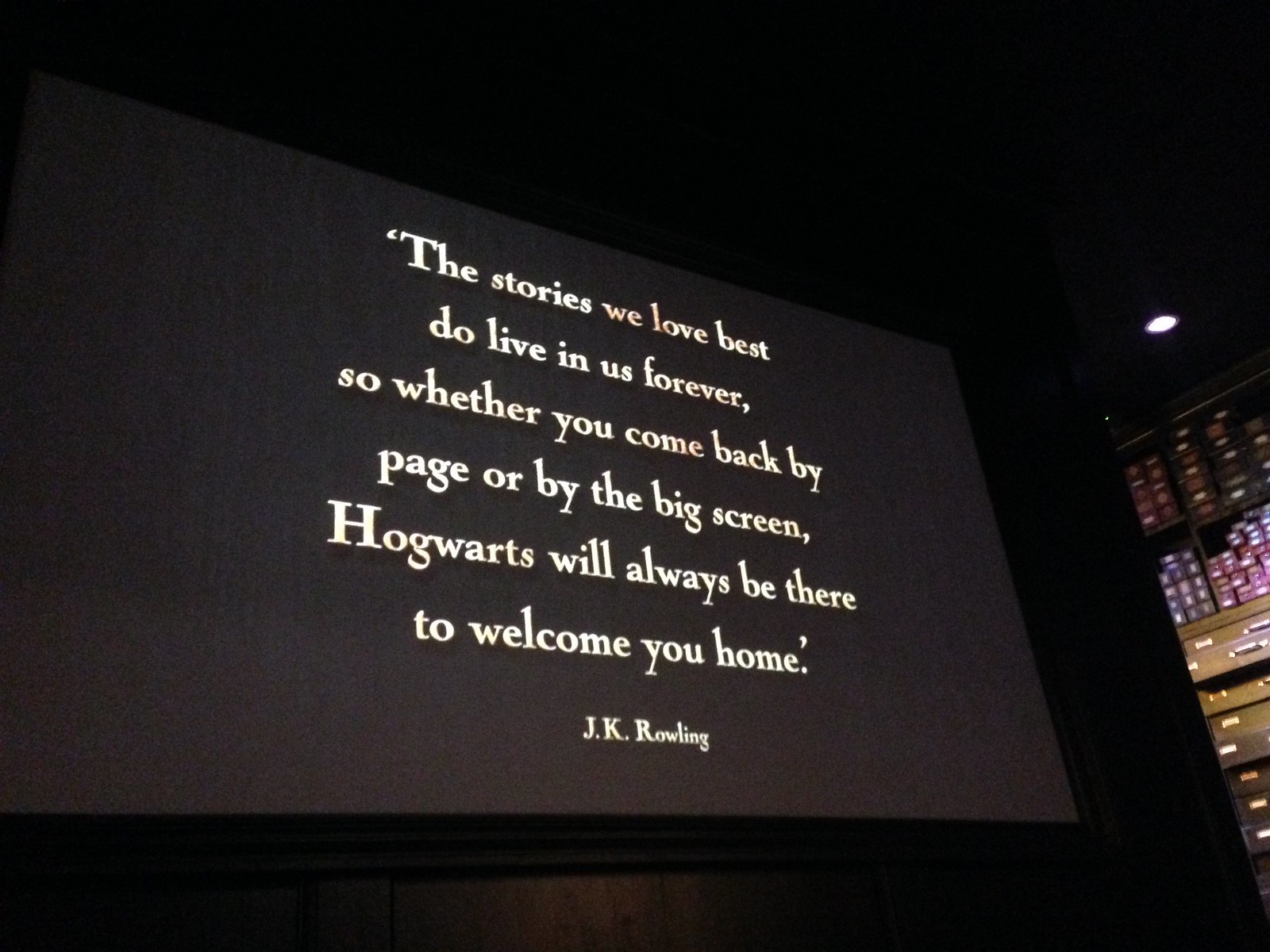The image is a color photograph in landscape orientation, capturing a movie theater screen from a slightly upward angle. The surrounding environment is dimly lit, with a noticeable single overhead light to the top right corner. On the right side of the photo, there are sliding shelves with numerous green drawers adorned with silver handles, and purple packages stacked in separate boxes.

The movie theater screen itself is black with several lines of text in bold, white lettering. The quote displayed reads: "The stories we love best do live in us forever, so whether you come back by page or by the big screen, Hogwarts will always be there to welcome you home." Below this heartfelt message, the author's name, J.K. Rowling, is prominently noted. The overall scene suggests this is the beginning of a Harry Potter movie screening, emphasizing the timeless and welcoming nature of the beloved Hogwarts world, whether experienced through books or movies.